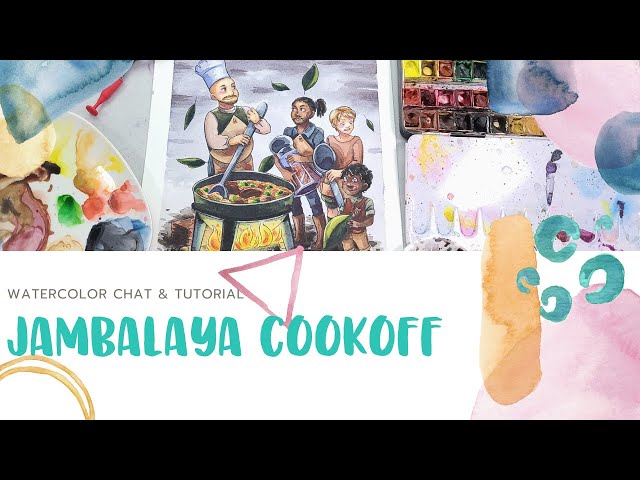The image is a detailed flyer or digital thumbnail, likely a screenshot from a YouTube video, titled "Watercolor Chat and Tutorial: Jambalaya Cookoff." The title "Jambalaya Cookoff" is prominently displayed underneath, with "Watercolor Chat and Tutorial" engraved above it. The design features a lower half with a white background, adorned with a light pink triangular pattern and golden ring motifs. The upper section consists of three watercolor illustrations:

1. The first panel depicts a large cast-iron pot on a fire, with a chef in a tall hat stirring it with an oversized spoon. The chef appears to be preparing jambalaya, surrounded by children holding large spoons and bowls, with leaves flying in the background.
2. The second panel showcases a painter’s palette with mixed paints and a painter’s box with multiple colors, suggesting an artistic theme.
3. The third panel contains a more abstract watercolor image, displaying ink bleeding into the paper with shapes like a pink triangle, a yellow rectangle, and a C-shaped form.

The overall aesthetic combines elements of cooking and watercolor art, creating a vibrant and engaging visual composition.